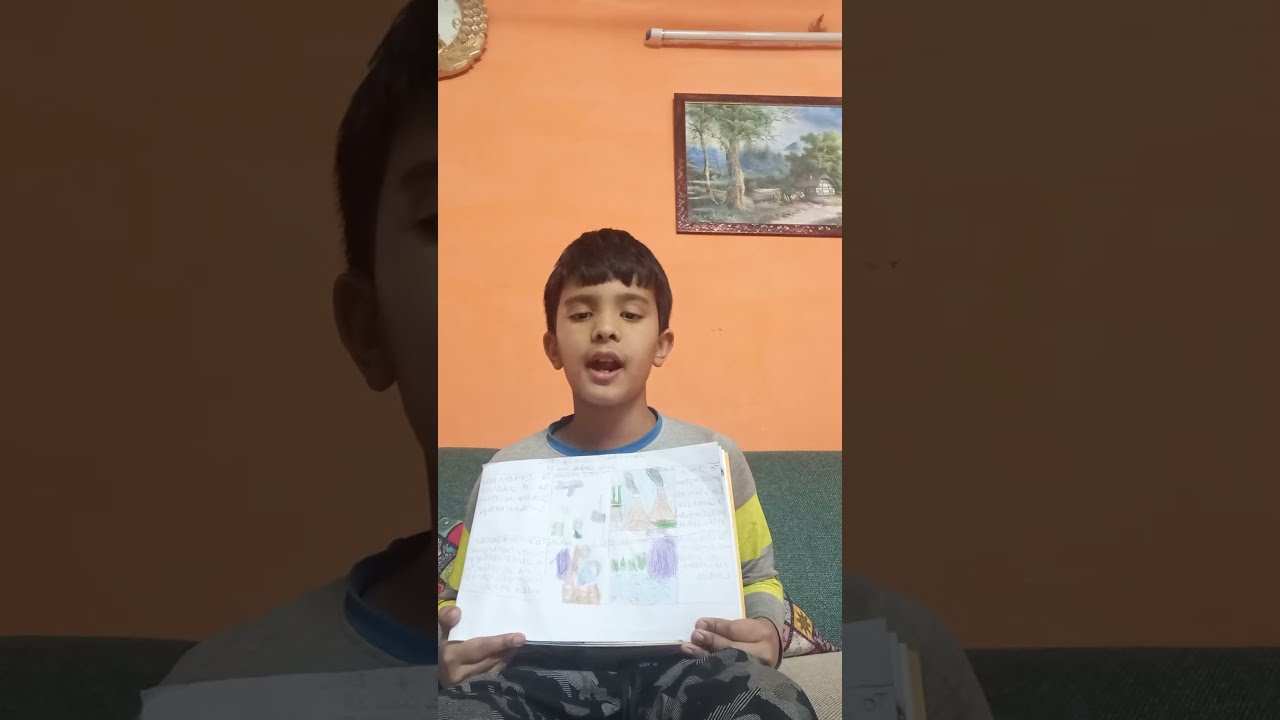In the photograph, a young boy sits on a couch holding up a piece of paper featuring his drawings and writing. He has short black hair and seems to be mid-sentence, gazing directly at the camera. He is dressed in a long-sleeved gray shirt with yellow stripes along the sleeves, blue trim around the collar, and gray camouflage-style pants. The backdrop consists of a light orange wall adorned with a mounted artwork, resembling a landscape with a house, a dirt driveway, and trees, lacquered onto a wooden surface. A white light bar or rod is positioned above the artwork, and there's a fragment of gold-colored ornamentation visible in the upper-left corner of the image. The photo utilizes a layered effect where a zoomed-in, blurred version of the image serves as the background, with the main image spliced into the center.